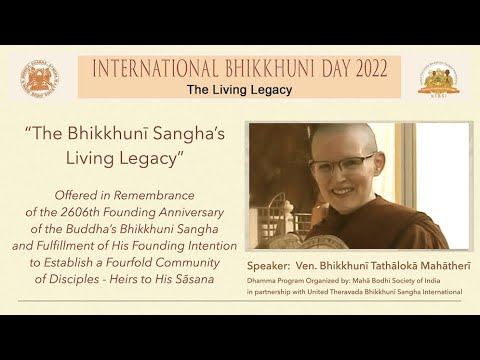This detailed landscape-oriented color photograph showcases a notice in celebration of International Bhikkhuni Day 2022. The words "International Bhikkhuni Day 2022" are prominently displayed in dark burgundy letters atop a peach-colored horizontal rectangle on a cream-colored background. Below, in smaller black text, it reads "The Living Legacy." Positioned centrally in the photograph is a smiling female Buddhist dignitary, identifiable by her shaved head, glasses, and dark burgundy robe. She is standing in front of a window, encapsulated by her serene ambiance. Her labeled caption, "Speaker: Venerable Bhikkhuni Kathalaka Mahathiri," appears below her image situated on the right side of the notice. The image also includes additional dark red text explaining the significance of the event: "offered in remembrance of the 2606th founding anniversary of the Buddha's Bhikkhuni Sangha and fulfillment of his founding intention to establish a fourfold community of disciples heirs to his sasana." Two circular logos flank the text arrangement, emphasizing the spiritual heritage being honored. The photo is bordered by black horizontal stripes both at the top and bottom, enhancing its design, which combines photographic realism with graphic design elements.